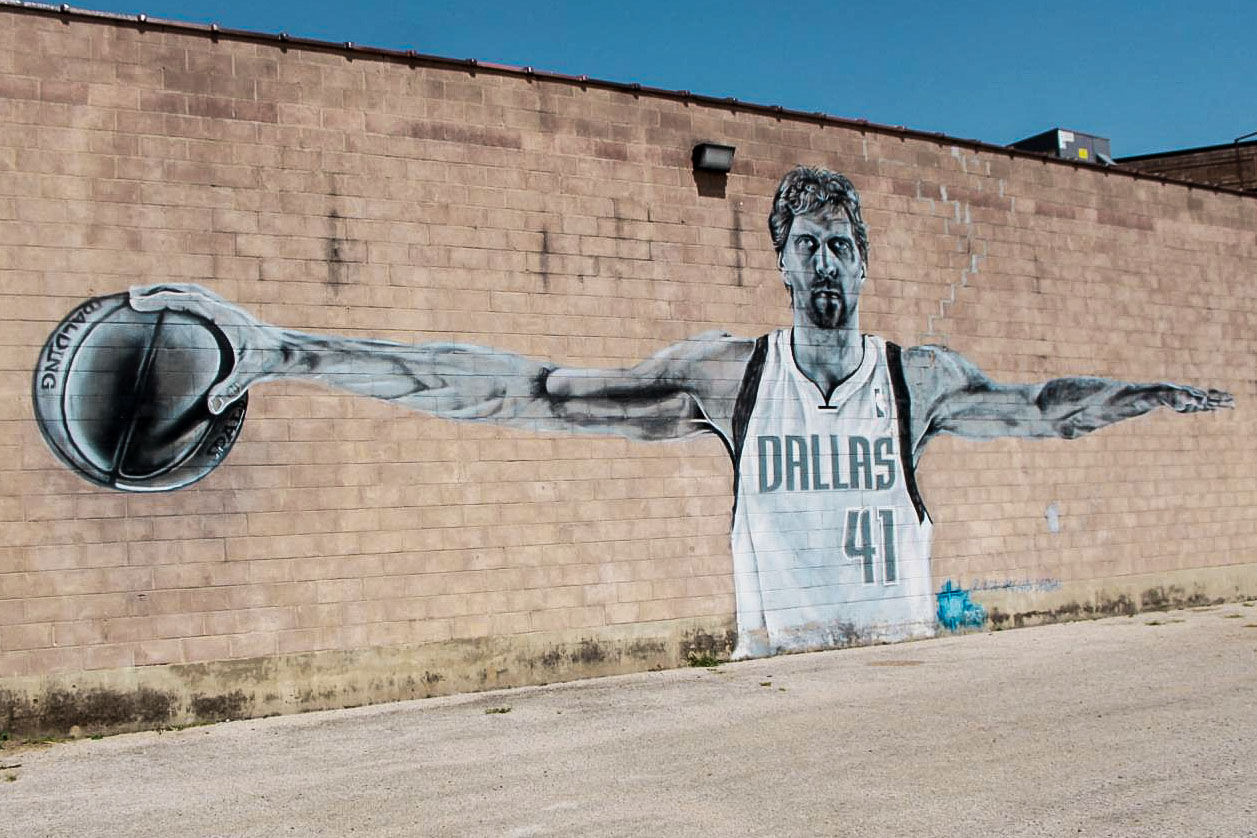The image features a detailed mural of Dirk Nowitzki, the renowned Dallas Mavericks player, painted on a somewhat stained and aged brick wall. The mural captures Dirk with his arms outstretched, wearing his iconic number 41 Mavericks jersey. The jersey, made distinct with large uppercase "DALLAS" lettering and the number 41 in gray and outlined in white, features the NBA logo on the top right. Dirk, depicted with a goatee and short, slightly shaggy hair, holds a basketball palming it in his right hand (left side of the mural), marked with "Spalding." Above the mural is a clear blue sky, and there's a light fixture at the top center of the wall, which adds to the mural’s prominence on the red brick building. The right side of the wall appears to recede slightly, indicating the angle of the shot.